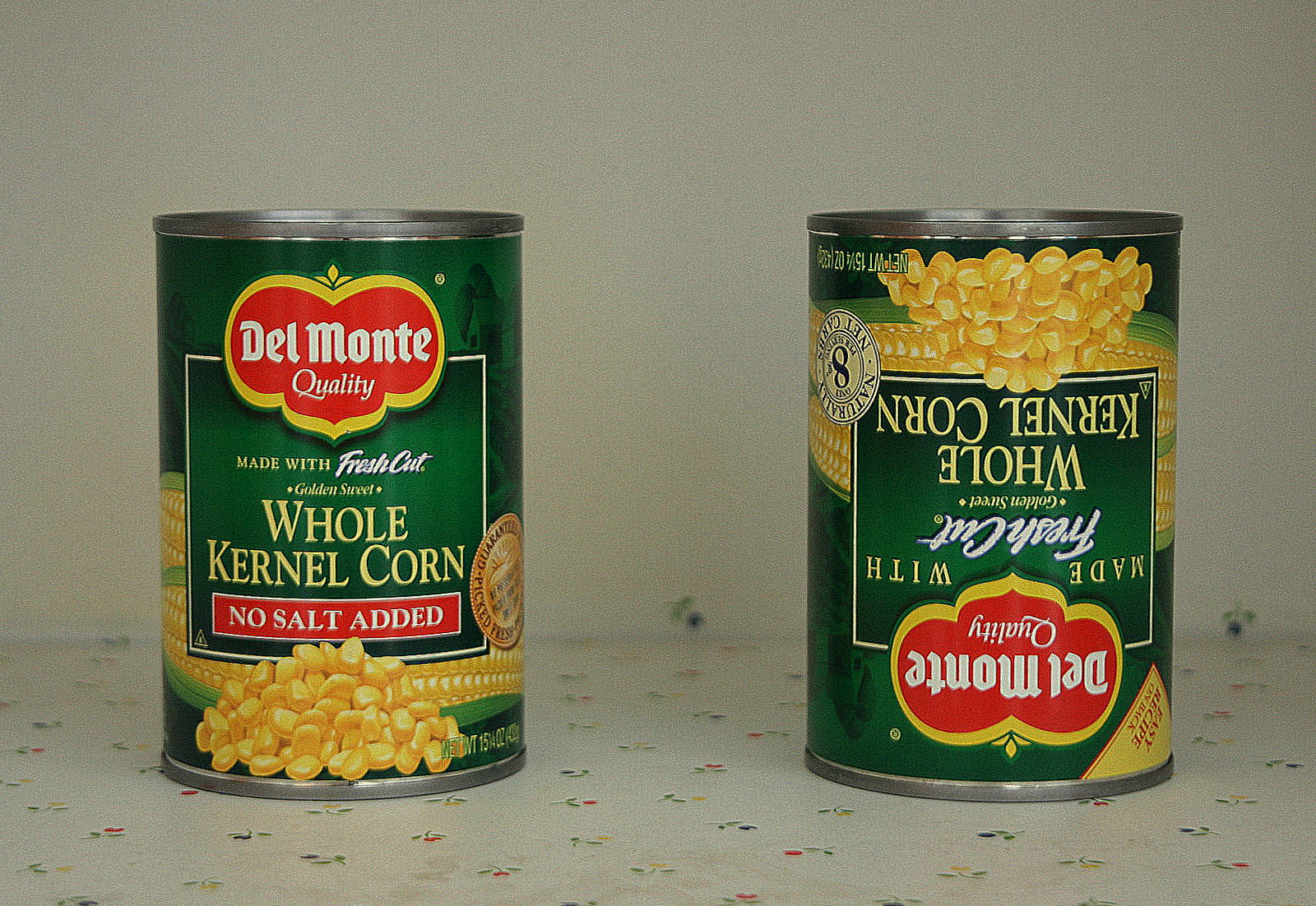The image displays two cans of Del Monte quality whole kernel corn on a table adorned with a white tablecloth featuring small flowers of various colors, including pink, yellow, and green. One can is upright, showcasing a label that reads "Del Monte Quality," with a yellow shield and red banner, underneath which it states "Made with fresh cut, whole kernel corn" in a green square. A red strip with white letters indicates "No salt added." The label includes an image of corn niblets in front of two corn cobs with green husks and a farm scene in the background. The second can, positioned next to it, is upside down, displaying the same Del Monte branding but without the "No salt added" mark. The table and the detailed floral tablecloth, against a white wall, set a subtle backdrop for the cans, one of which bears an additional unreadable emblem and mentions "easy recipe" in a corner.